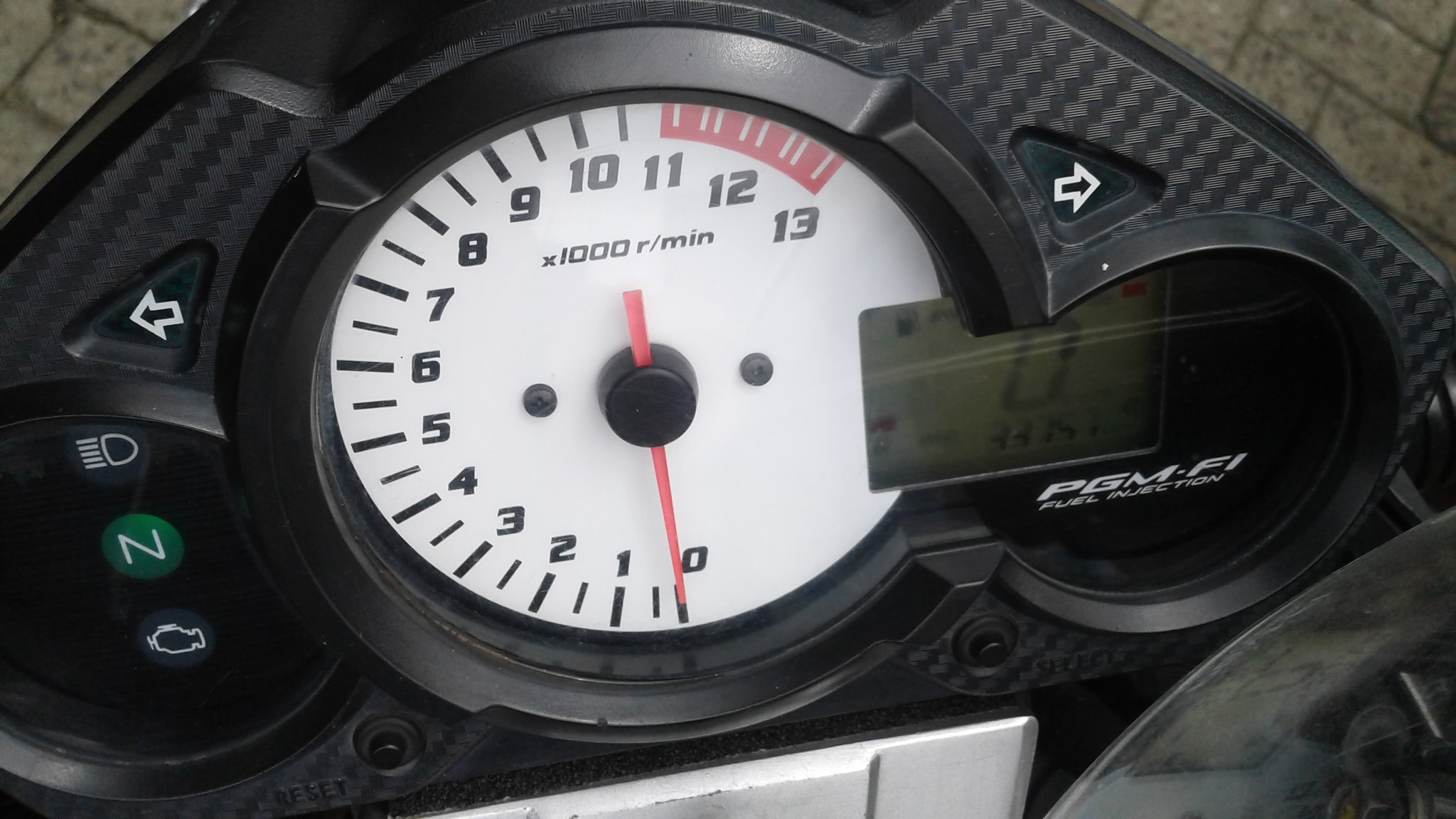The image captures a detailed close-up of a vehicle's dashboard, which likely belongs to a motorcycle, moped, or electric bike. The photograph is taken from a perspective that includes portions of the gray brick pavement in the top left and top right corners.

The dashboard display is encased in plastic. Dominating the center is a large, white analog RPM gauge. The gauge ranges from 0 at the bottom to 13 at the top right, with the numbers 11, 12, and 13 highlighted in a white font within red boxes. A red needle on this RPM gauge currently points to 0. Above the needle, the label "X1000R/MIN" is clearly visible. Flanking the RPM gauge are indicators for the right and left turn signals.

To the right of the RPM gauge is a digital screen, displaying a prominent "0," likely indicating speed, among other functions that aren't entirely distinguishable in the image. The screen also features the acronym "PGM."

On the left side of the RPM gauge, there is an array of indicator lights. One light features a high beam symbol within a gray circle, another shows a green "N," and a third presents an engine symbol within a gray circle.

This detailed dashboard setup provides essential information for the rider, including RPM, speed, and various operational indicators.